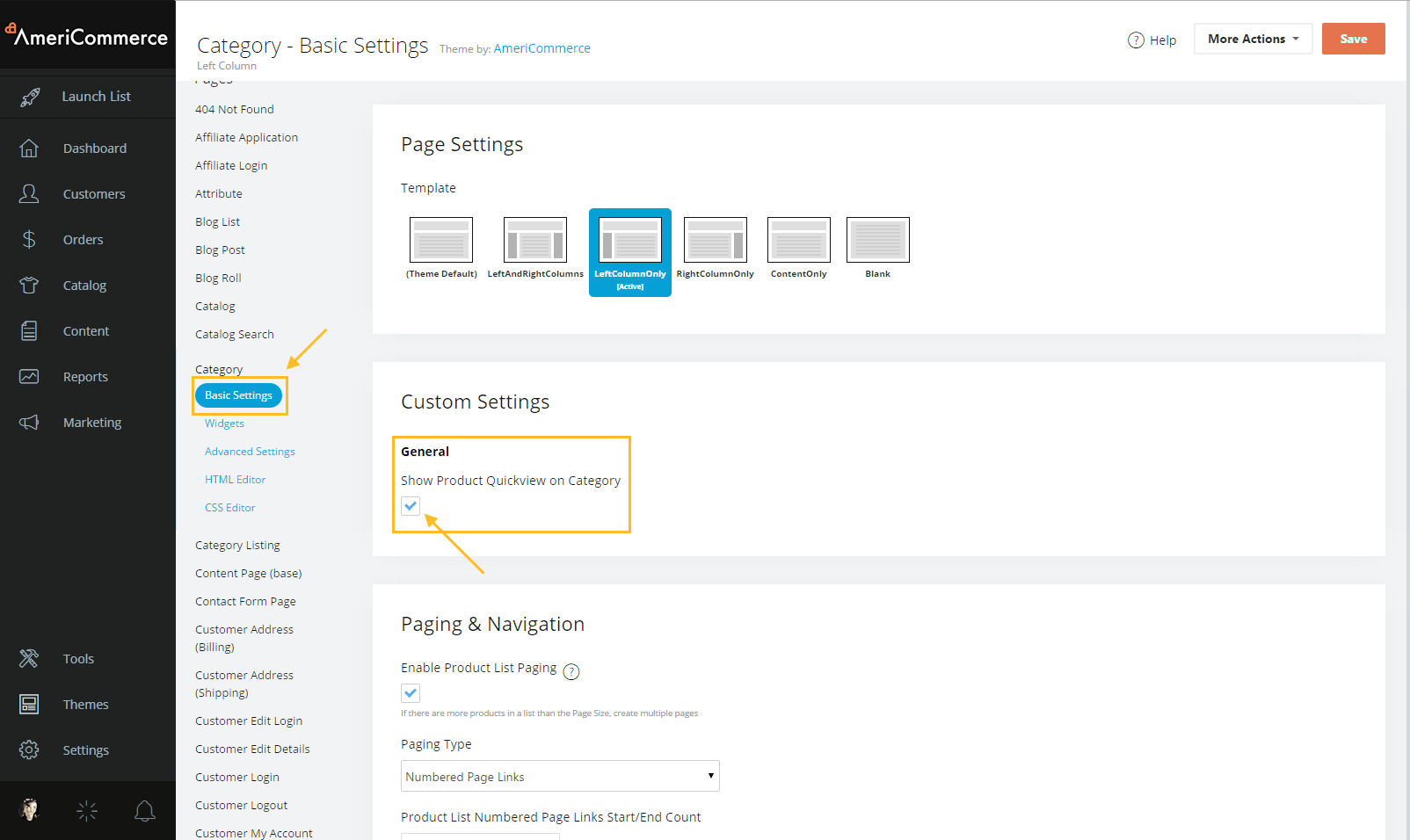This image is a screen capture of the AmeriCommerce website or application interface. On the far left, there is a vertical menu column featuring a black and dark gray background with white text. At the very top of this column, it displays the label "AmeriCommerce" accompanied by an icon resembling a sideways heart. The menu is divided into two sections. The upper section includes the following options, each with a corresponding icon: Launch List, Dashboard, Customers, Orders, Catalog, Content, Reports, and Marketing. The lower section lists Tools, Themes, and Settings.

The majority of the page exhibits a white and gray color scheme. At the top, under the category "Basic Settings," the heading "Theme by AmeriCommerce" is visible. Various page setting templates are displayed, offering different customization options alongside settings and navigation configurations.

To the right of the primary content area, there is a secondary menu column. This column includes text entries such as "404 Not Found," "Affiliate Application," "Affiliate Login," "Attribute," "Blog List," "Blog Post," and "Blog Roll," among others, providing additional navigational options within the application.